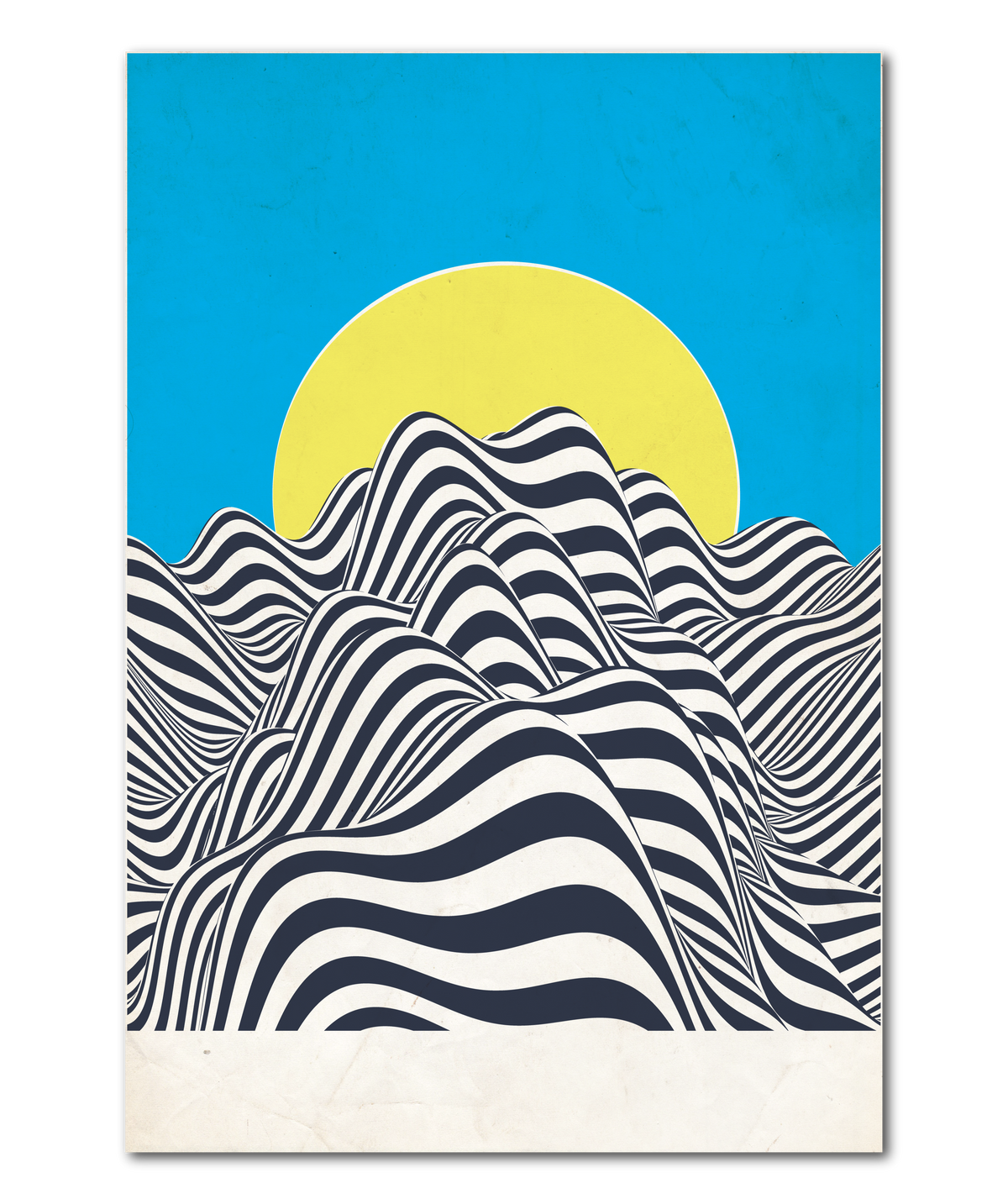This rectangular artwork, measuring approximately 5 inches high by 3 inches wide, features a striking black and white wavy pattern reminiscent of zebra stripes, occupying the lower half of the image. At the bottom of this wavy design is a plain white footer, extending upward about half an inch. Rising behind this wavy pattern, a yellow sun with a thin white outline sits at the center, partially covered by the black and white waves. The background showcases a serene blue sky, with subtle indications of clouds staining the upper section of the image from left to right. A slight gray shadowing is visible along the right-hand side of the picture, stretching from the top right corner to the bottom, adding depth to the composition. The detailed interplay of these elements creates a visually dynamic scene that is both intriguing and harmonious.